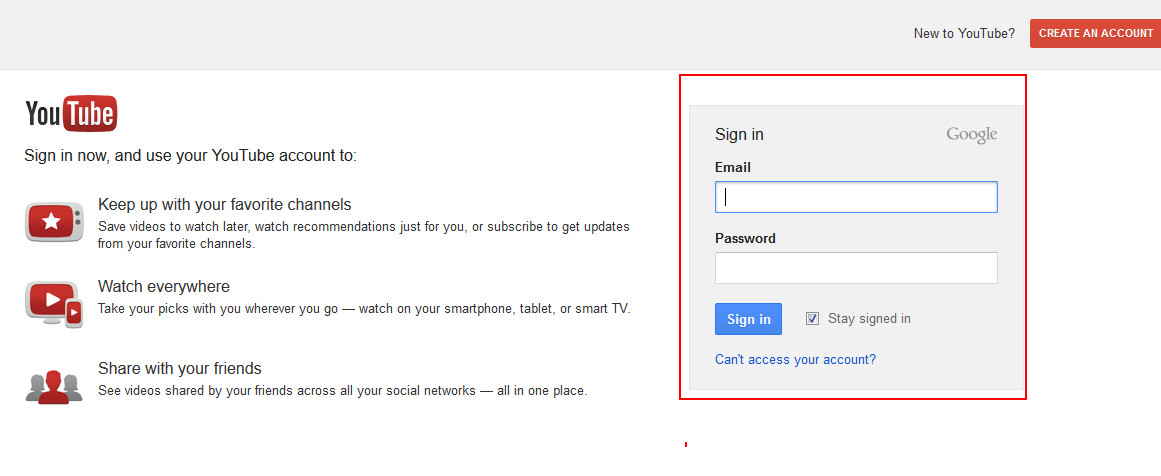This color photograph appears to be a screenshot from a YouTube web page inviting new users to create an account or sign in. In the top right corner, there's a prompt that reads "New to YouTube?" in black with a question mark at the end. Directly below, a white "Create an account" link is highlighted with a red border. Below this section, there is another interactive area for existing users to sign in through Google. This section features a red-bordered "Sign in" button, accompanied by text fields for "Email" and "Password." Below these fields, a blue "Sign in" button is prominently displayed, along with a checkbox option to "Stay signed in."

Further down, there's a hyperlinked question, "Can't access your account?" providing help for users struggling with passwords or usernames.

On the left side of the page, there is informational text encouraging users to sign in to YouTube. It elaborates on the benefits of having an account, such as keeping up with favorite channels, saving videos to watch later, receiving personalized recommendations, and subscribing for future updates. The information also highlights the versatility of accessing YouTube on various devices, including smartphones, tablets, and smart TVs, and mentions the ability to share videos across social networks. This comprehensive layout aims to guide users smoothly through account creation or sign-in to enhance their YouTube experience.